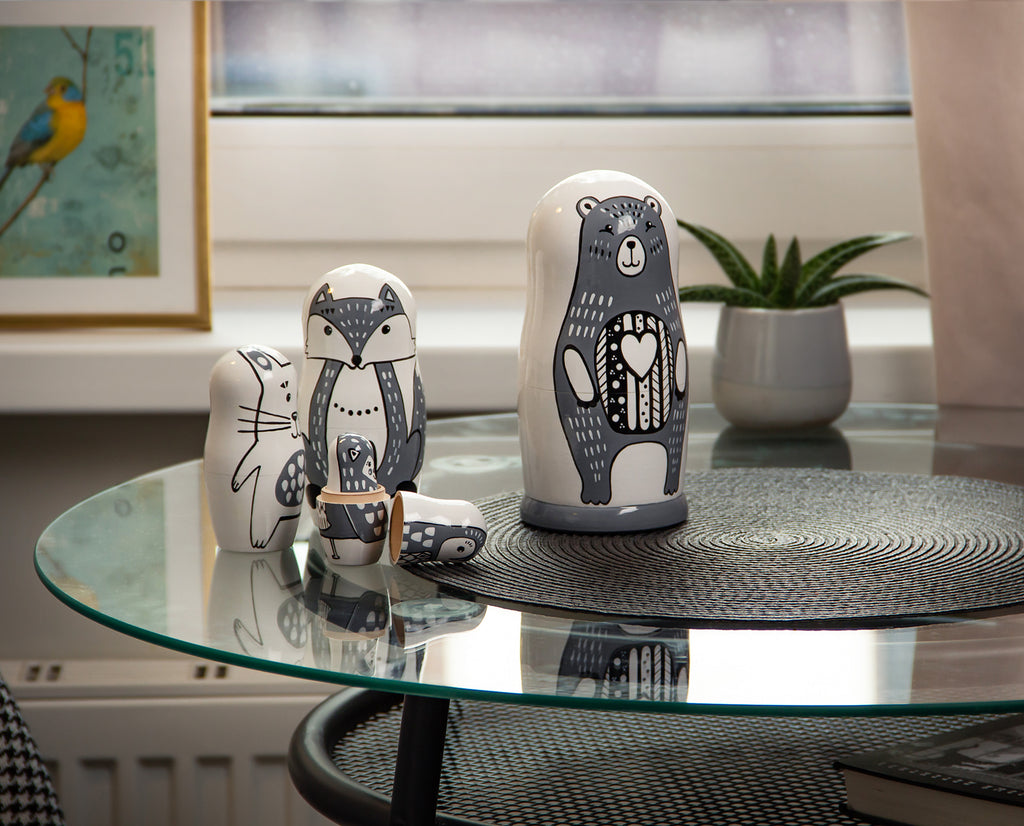The photograph, taken indoors, centers on a glass-topped coffee table. The table, rectangular in shape and measuring roughly five by six inches, features a metal grid pattern visible underneath the glass. Positioned atop this glass surface is a small, round place setting, situated centrally. Alongside it, on the left side, stands an oblong, gray-based statue embellished with a white backdrop and an illustration of a large gray bear with a heart on its chest. 

Adjacent to the bear statue, there are smaller stacking dolls, each fitting within the other. The second largest doll displays a gray fox painting, followed by a smaller rabbit doll to its left. In front of these, one doll has its top resting sideways, revealing a tiny bird-like figure inside with an even smaller doll nested within it. 

In the room's background, a white potted plant with long green leaves is visible on the right. The background wall is white, adorned with a radiator at the bottom and a window higher up, through which gray light filters. To the left of the window, a framed picture showcases a bird with vibrant yellow plumage on its chest and blue wings. On the right-hand side of the window hangs a light pink curtain. A hardback book sits partially visible beneath the glass tabletop on the bottom metal grid.